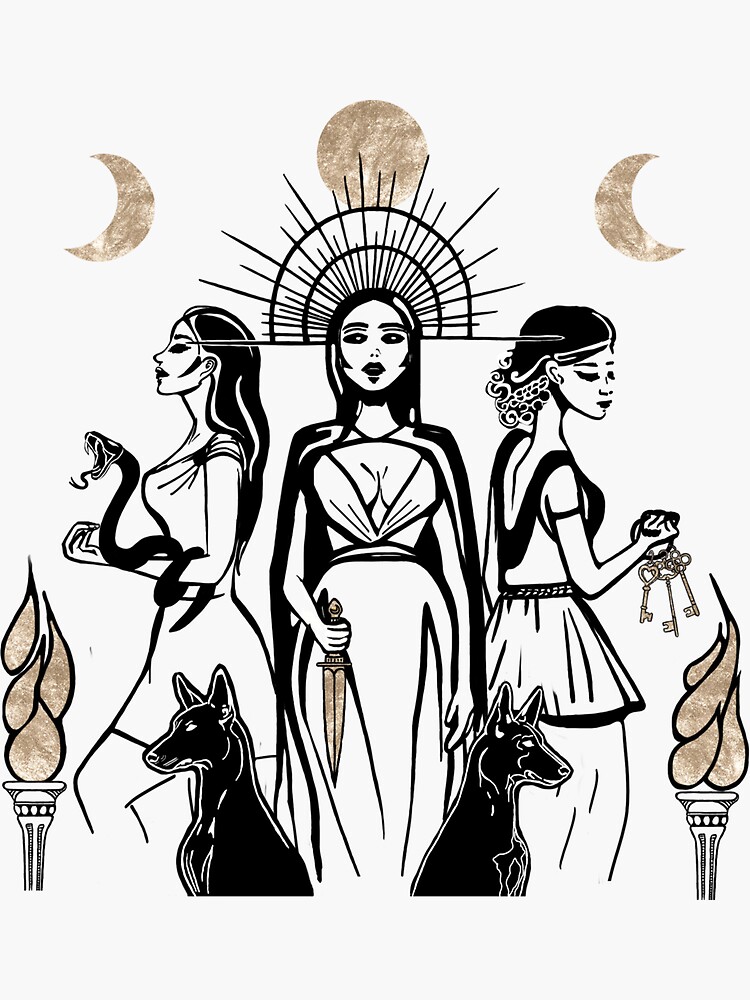The image is an intricately detailed black and white drawing set against a white background, accented with gold highlights. At the top, it features a sequence of three moons: a gold crescent moon facing left on the top left, a full gold moon in the top middle, and another gold crescent moon facing right on the top right. Below these celestial elements, the center of the image showcases three Egyptian-inspired women.

The leftmost woman is depicted from a left-side view, featuring long black hair and a black snake coiled around her arm with its mouth open. The central figure wears a white dress with black outlines and is adorned with a black cape. She wields a gold dagger pointed downward in her right hand and wears a distinctive crown resembling a half-circle with lines radiating out like sun rays. The woman on the right, viewed from her right side, mirrors the central figure's attire—a white dress with black accents—and holds a set of gold keys in her right hand. She has short black hair and is gazing downward.

Accompanying these women are two black dog-like figures, possibly representing Egyptian deities, positioned at the bottom center. On either side of these canine figures are torches with gold flames, contributing to the image's symmetrical balance and the mystical ambiance. Overall, the image combines mythological motifs with a striking use of contrasting colors and intricate line work.